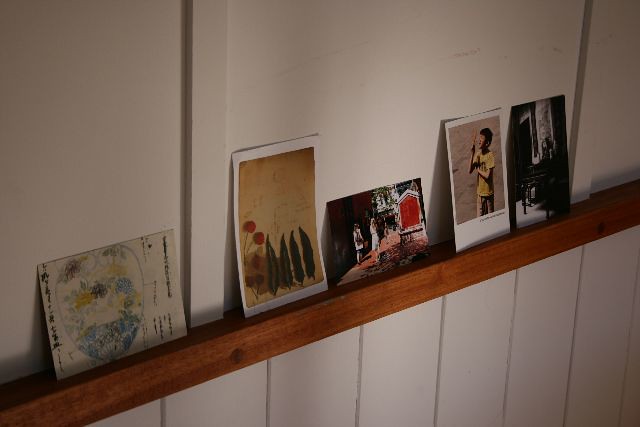This image showcases a section of an interior wall adorned with a wooden chair railing, which is home to a collection of five small, postcard-like pavers, possibly photographs or cards. The chair railing is a thin horizontal strip of wood separating the white wall above and a panel of vertical rectangular white strips below. The postcards vary in orientation and content:

1. The first postcard on the left is wider than it is tall and appears to feature a low-resolution drawing with a circular design and plant-like elements, possibly accompanied by Japanese text.
2. The second card is distinguished by its white border and depicts trees or peppers at the bottom and a flower in the bottom left corner, set against a light brown background.
3. The third item appears to be a photograph capturing an outdoor scene with two girls surrounded by pink and red hues, standing next to a red building. 
4. The fourth is a Polaroid photograph of a boy in a yellow shirt and either small green shorts or brown pants, with a brown, possibly dusty, background.
5. The fifth and final postcard is a black-and-white image that seems to feature a classic car, though the resolution makes it hard to discern the details clearly.

The overall composition blends the rustic charm of wooden elements with the nostalgic feel of displayed memorabilia.